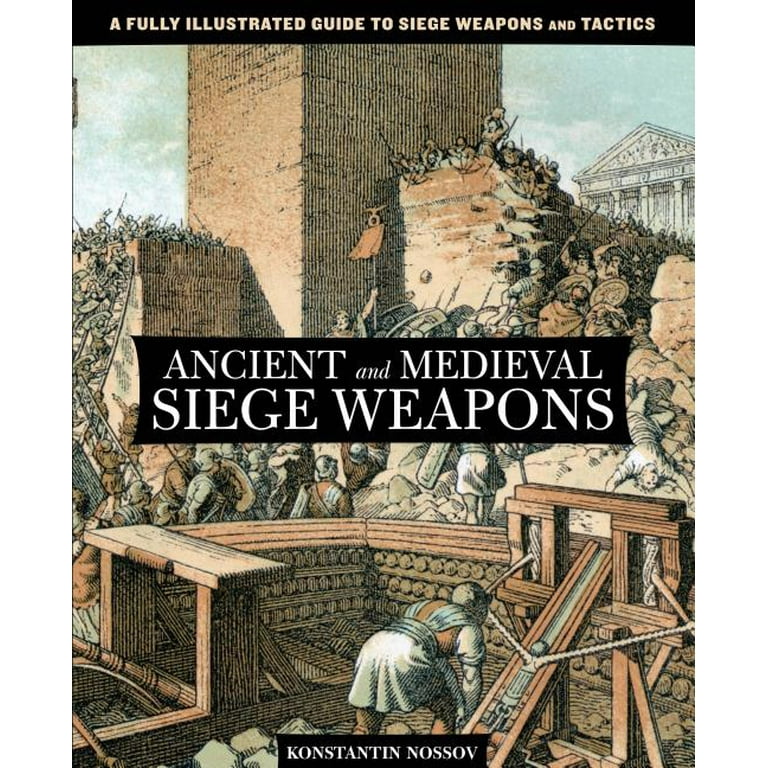The cover of the book "Ancient and Medieval Siege Weapons: A Fully Illustrated Guide to Siege Weapons and Tactics" by Konstantin Nesov features a detailed and colorized drawing depicting a chaotic medieval battle scene. In muted rust and blue-gray tones, the image shows an intense confrontation at a crumbling wall where one army is attempting to breach the defenses while the defenders fight from above. A catapult is prominently aiming at the wall, symbolizing the siege weaponry focus of the book. Soldiers below are scaling the wall with ladders while rocks and other projectiles are launched down at them by the defenders. Some men lie on the ground, possibly wounded or dead, while others with shields continue the fight. In the background, a classical temple-like structure adds to the historic ambiance. One soldier is seen holding a flagpole, possibly signaling the act of claiming territory in the midst of the battle. The title is clearly centered, emphasizing the book’s focus on the weaponry and tactics of ancient and medieval warfare.